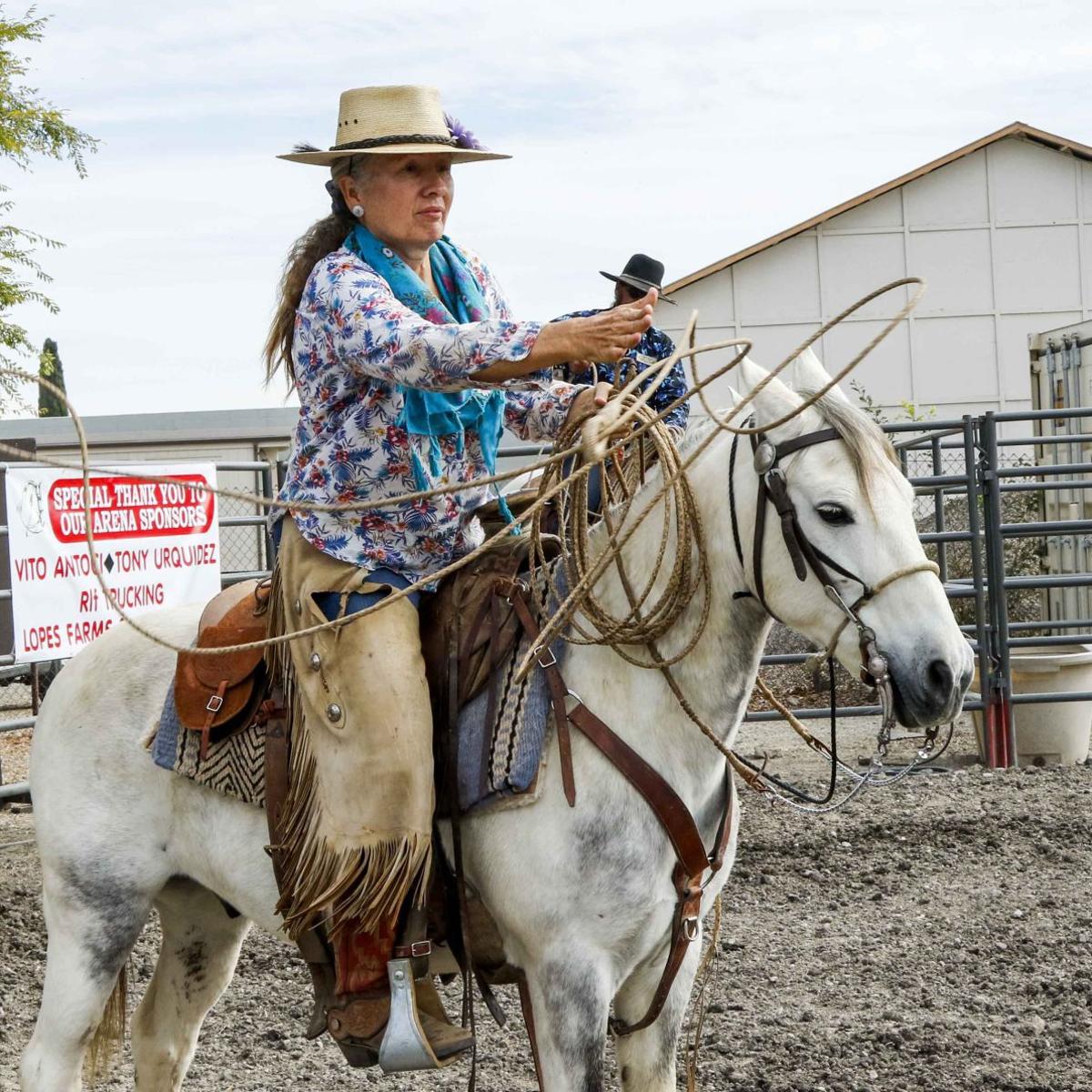In this image, a middle-aged woman of possible Indian heritage is riding a white horse with a black snout and mane. The woman has long gray hair tied in a ponytail and wears a stylish straw hat adorned with a dark brown band and a purple flower. Her outfit includes a colorful floral shirt with a mix of blue, red, and pink petals, and a turquoise scarf that features additional floral patterns. She dons cowboy chaps fringed on the outer edges, brown boots, and wields a brown rope in her hands as if preparing to lasso.

Beneath her brown leather saddle lies a woven Navajo-pattern blanket in shades of purple, white, and black, designed to enhance the horse's comfort. The scene is set in a dusty arena surrounded by a metal fence. In the background, there's a white building with a pitched roof and a partially visible tree with green leaves. The cloudy sky above creates a serene backdrop.

To the left of the image, a bilingual sign reads "Special Thank You to Our Arena Sponsors" in both English and Spanish, printed on a white and red banner. Additionally, there's a man wearing a black cowboy hat standing behind her, possibly an instructor assisting her in the arena. The overall setting is a horse pen filled with brown dirt, framing the dynamic moment of her riding experience.